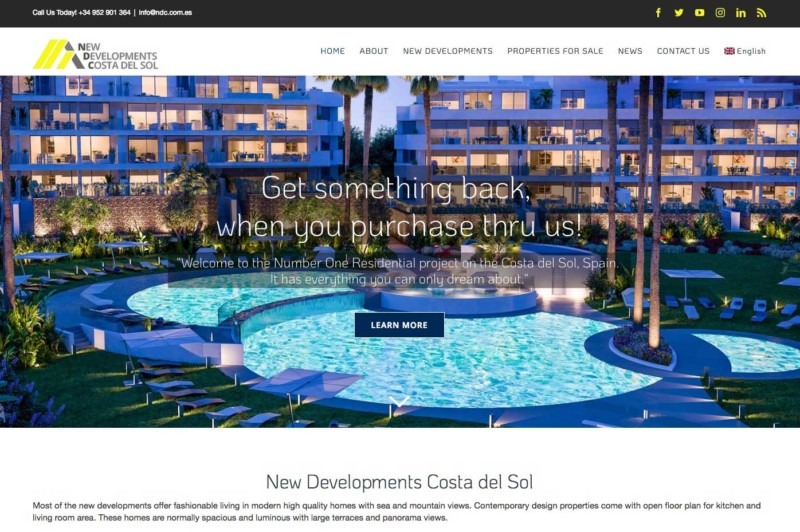This image depicts the homepage of the real estate website "New Developments Costa Rica Del Sol." The website's top section features contact information with a prompt to "Call us today" at +34-952-001364 or email at info@ndc.com.es. Social media icons for Facebook, Twitter, Instagram, YouTube, LinkedIn, and an RSS feed are also prominently displayed.

The navigation menu includes options such as Home, About, New Developments, Properties for Sale, News, and Contact Us, with the language setting set to English. The main content highlights a large header image showcasing a modern residential development, complete with a luxurious swimming pool surrounded by lush palm trees. A text overlay reads, "Get Something Back When You Purchase Through Us. Welcome to the number one residential project on the Costa Del Sol, Spain. It has everything you can only dream about." A prominent "Learn More" button sits in the center of the image.

Below the header image, a section titled "New Developments Costa Del Sol" offers a brief description of the available properties. It emphasizes the quality homes, contemporary design, open floor plans, large terraces, and panoramic views. The luxurious swimming pool mentioned earlier adds to the allure, making it a focal point of interest.